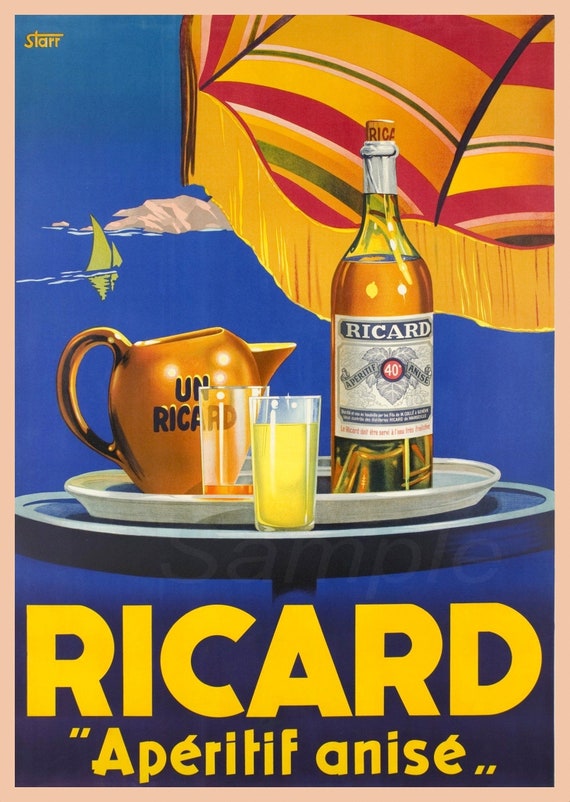This vintage advertisement poster, likely from the 1940s or earlier, is a painted illustration promoting "Ricard Aperitif Anise." The centrally featured Ricard bottle, with its gold-brown label, is elegantly positioned on a platter atop a table, which appears to be suspended in mid-air over a sea-like, blue background. Below the bottle, the bold yellow text reads "Ricard Aperitif Anise."

Accompanying the bottle on the platter are two glasses: one containing a golden-colored liquid, presumably the advertised anise aperitif, and the other with a nearly empty serving of what seems to be orange juice. Partially visible in the top right corner is a striped umbrella in shades of orange, yellow, green, red, and white. To the left side of the image, a small, minimalistic green sailboat is seen sailing towards the right, against a backdrop of rocky cliffs. A golden image, labeled "Un Ricard," is also notable within the advertisement.

The entire composition exudes a nostalgic charm, enhanced by its peach border, classic visual elements, and serene seaside atmosphere, capturing the essence of vintage advertising artistry.